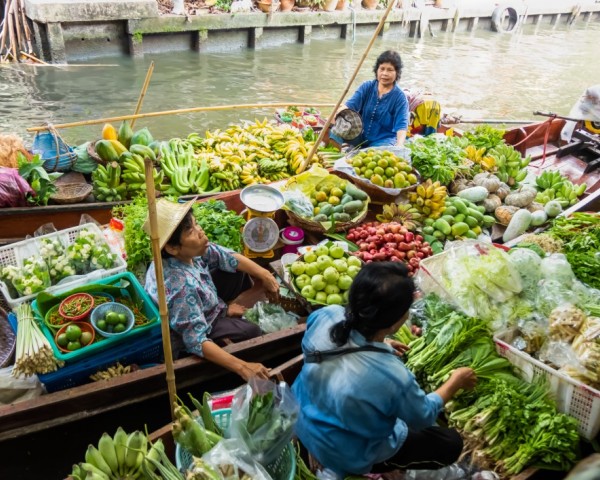The image depicts a vibrant floating market scene, likely set in Southeast Asia, where three canoe-like boats brimming with a variety of fruits and vegetables are arranged in a picturesque waterway against the backdrop of an outdoor storefront. In the topmost boat, a woman with short black hair, clad in a blue shirt, navigates alongside the dock. This vessel is laden with bananas and other produce. The central and largest boat features a man with a light-colored hat and a blue patterned shirt, focused on his vegetable scale, his arms reaching out to the neighboring boat. His boat carries a colorful array of apples, pears, limes, peppers, and assorted fruits. The bottom boat, positioned closest to the viewer, contains a woman with long black hair tied back, wearing a light blue shirt and dark pants, steering amidst a bountiful cargo of bananas, papayas, and leafy greens. The collective imagery captures the bustling energy and rich cultural tapestry of a floating market teeming with life and fresh produce, framed by the water and the rustic charm of the storefront.